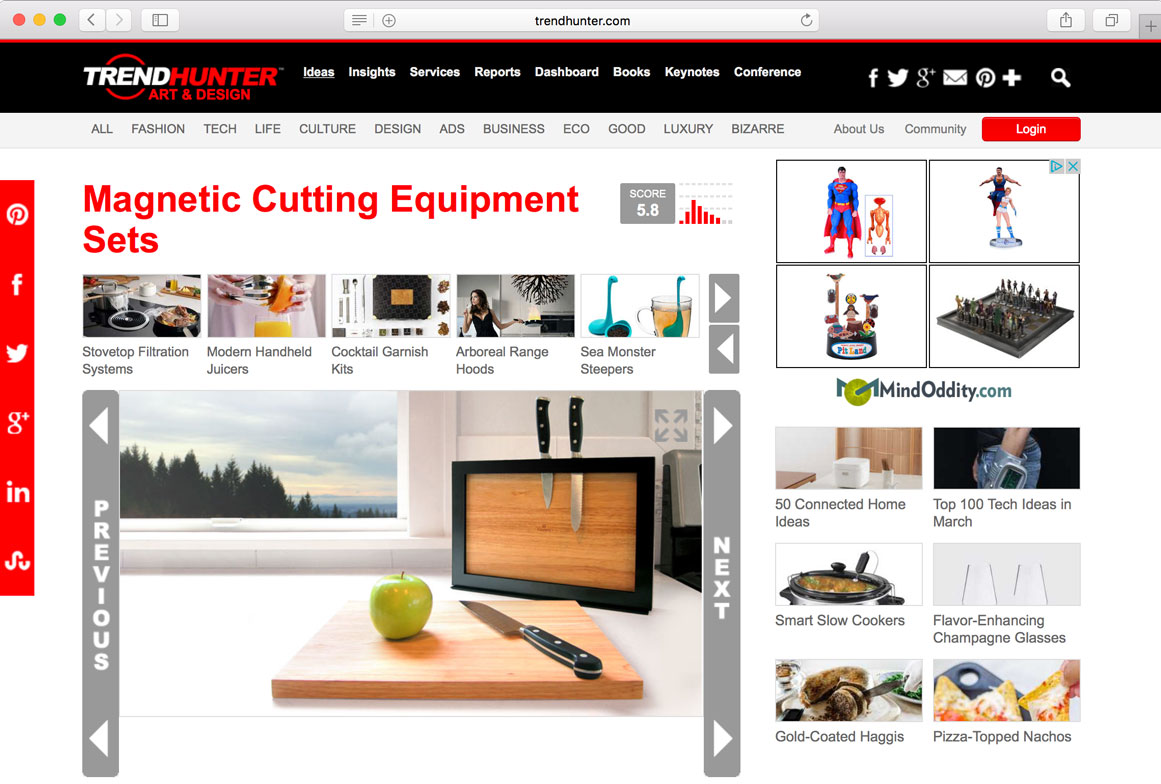This image displays a detailed screenshot of a website named Trend Hunter Art and Design. 

At the top, there is a gray rectangular section showing the upper portion of the website interface. Below it is a black rectangular strip stretching horizontally across the page, prominently featuring the name "Trend Hunter Art and Design". On the right side of this strip, the navigation options include "Ideas," "Insights," "Services," "Reports," "Dashboard," "Books," "Keynotes," and "Conference." Additionally, social media icons are available for easy sharing, along with a search bar for more precise navigation.

Directly beneath this section, the categories listed are "Awe," "Fashion," "Tech," "Life," "Culture," "Design," "ADS," "Business," "Eco," "Good," "Luxury," and "Bizarre." There are also links for "About Us" and "Community."

The central part of the image features a large picture advertising "Magnetic Cutting Equipment Sets." The image showcases an apple placed on a cutting board, with a knife positioned beside it. In the background, it highlights the magnetic feature that allows knives to be attached to the board. Adjacent to the image is a score of 5.8 accompanied by a bar graph.

Additional items displayed on the right side of the page include Halloween costumes and chess boards, among other products.

This detailed caption aims to provide a comprehensive visual description of the website's layout and content.